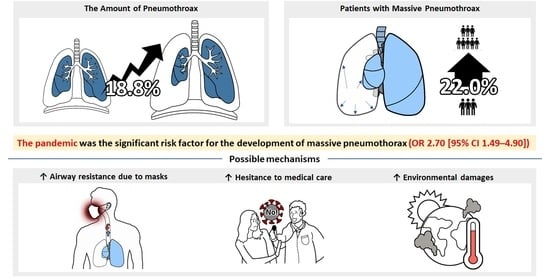The illustration is a detailed medical and scientific diagram on a white background, featuring various drawings in black, with some parts highlighted in blue and red. At the top of the diagram, there is bold text stating "The pandemic was a significant risk factor for the development of massive pneumothorax," accompanied by the statistical notation (OR 2.70 [95% CI 1.49 to 4.90]). The upper section is divided into two smaller diagrams: one showing a pair of lungs with an arrow indicating an increase of 18.8%, labeled "The amount of pneumothorax," and another noting a 22.0% rise in "Patients with massive pneumothorax." 

Beneath these primary visuals, a longer diagram spans the width of the shorter ones above, presenting three small illustrations labeled "Possible Mechanisms." From left to right, these are: "Airway resistance due to masks," depicting partially obstructed lungs; "Hesitance to medical care," showcasing a slight delay in seeking medical attention; and "Environmental damages," illustrating external factors exacerbating health conditions during the pandemic. The diagram meticulously details the increase in pneumothorax cases and the potential causes linked to pandemic-related factors.